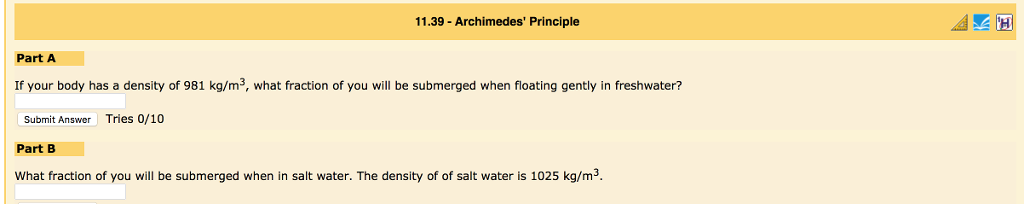A detailed caption for the described image would be:

---

The screenshot displays an educational interface on the topic of Archimedes' Principle, specifically curated for problem-solving exercises. The upper section of the interface features a prominent yellow bar, occupying approximately one-sixth of the page's height. This bar includes the title "11.39 Archimedes' Principle" in black text on the left, and three clickable sections on the right-hand corner for additional options or navigation.

Below this header, the interface presents two parts of a question (Part A and Part B), each pertaining to buoyancy in different water types. 

Part A, highlighted by a yellow background with black text, asks: "If your body has a density of 901 kg/m³, what fraction of you will be submerged when floating gently in fresh water?" A submission box and a status section indicating "Try 0 out of 10" accompany this question.

Part B, also highlighted in yellow with black text, inquires: "What fraction of you will be submerged in salt water with a density of 1025 kg/m³?" 

The overall page background is a tan color, providing a neutral backdrop for the yellow sections and ensuring high readability of the black text.

---

This caption encompasses all the visual and textual elements described, giving a reader a vivid and comprehensive understanding of the image.